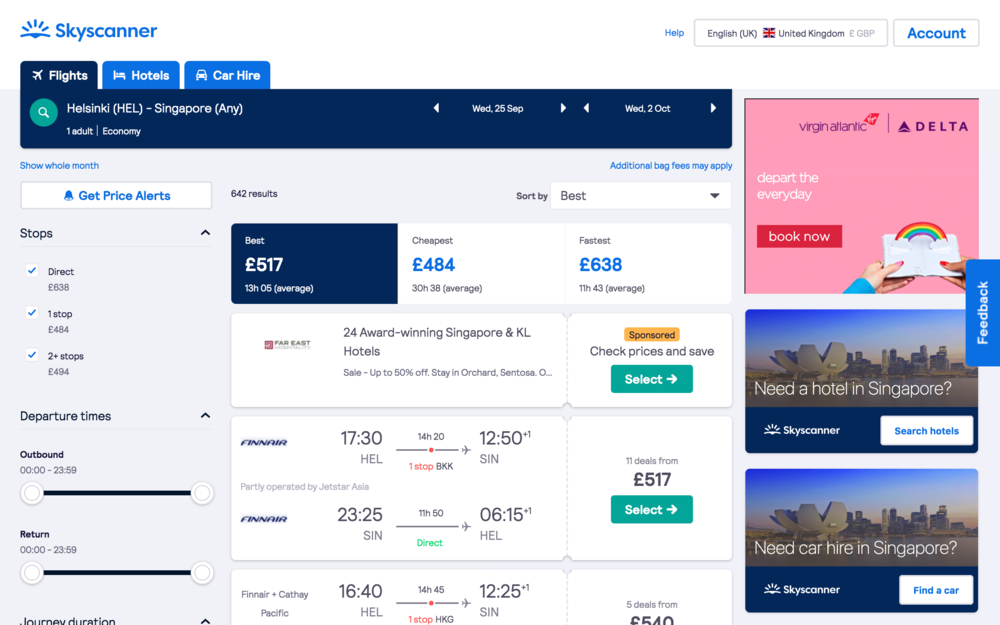This is a detailed screenshot of the flight search results page from Skyscanner, an online travel booking platform. At the top left corner of the webpage, the Skyscanner logo is prominently displayed, signifying the brand. To the right on the same row, options such as "Help," a small search bar, language selection displaying "English (UK)" with the United Kingdom flag, and an "Account" button in blue text are available.

Beneath the Skyscanner logo, there are four main tabs with "Flights" being the active tab. The search query is set for a round trip from Helsinki to Singapore, departing on Wednesday, 25th September, and returning on Wednesday, 2nd October. The search filters specify one adult traveling in economy class, yielding 642 flight options, which are sorted by the "Best" criteria.

Highlighted at the top are key options: the best option priced at £517, the cheapest option at £484, and the fastest flight lasting approximately 11 hours and 43 minutes priced at £638. Different selections based on flight duration and price are available for comparison.

Among the flight options, a sponsored selection from Far East features prominently, advertising 24-hour, award-winning Singapore and Kuala Lumpur hotels with a call-to-action button "Check prices and save."

Details of specific flights include:
- A Finnair flight departing from Helsinki at 7:30 PM (19:30) military time, reaching Singapore after 14 hours and 20 minutes with one stop.
- A return Finnair flight departing from Singapore at 11:25 PM (23:25) military time, arriving in Helsinki at 6:15 AM with a duration of 11 hours and 50 minutes for a direct flight, priced at £517. There are 11 deals available with a green "Select" button.

On the right side of the flight chart, there are three ad banners:
1. An advertisement from Delta Virgin Atlantic with a pink background, featuring an envelope with a rainbow emanating from it and a red "Book Now" button.
2. An ad asking, "Need a hotel in Singapore?" displaying the Singaporean skyline and offering a "Search hotels" button in white.
3. Another ad questioning, "Need a car in Singapore?" showing the same skyline and featuring a "Find a car" button, both ads from Skyscanner.

This detailed screenshot provides a comprehensive look at the layout, available options, and supplementary advertisements on the Skyscanner flight search results page.